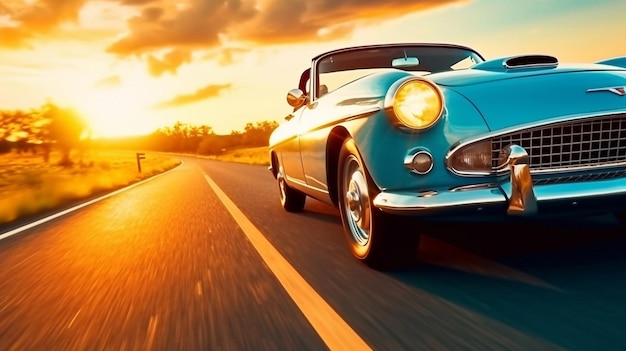The image features a vintage, sporty-looking blue car positioned on a road with distinctive round headlights and chrome details, including a logo or possibly a "T" on the front. The scene is set at an angle, showing the car in front of a dramatic backdrop. The sky is a mix of light blue with dark clouds at the top of the frame, and a brilliant sunset that casts a golden hue over everything. The road stretches out ahead with a prominent yellow line down the middle, flanked by white lines on either edge. On either side of the road, there are trees and patches of grass, contributing to the picturesque, natural setting. The front top light of the car is lit in orange, adding a further touch of vintage charm. Overall, the image exudes a warm, nostalgic feel with the sun glowing bright yellow in the top left, trees lining the road, and a serene mix of golden sunlight and shadows enhancing the car's classic appeal.